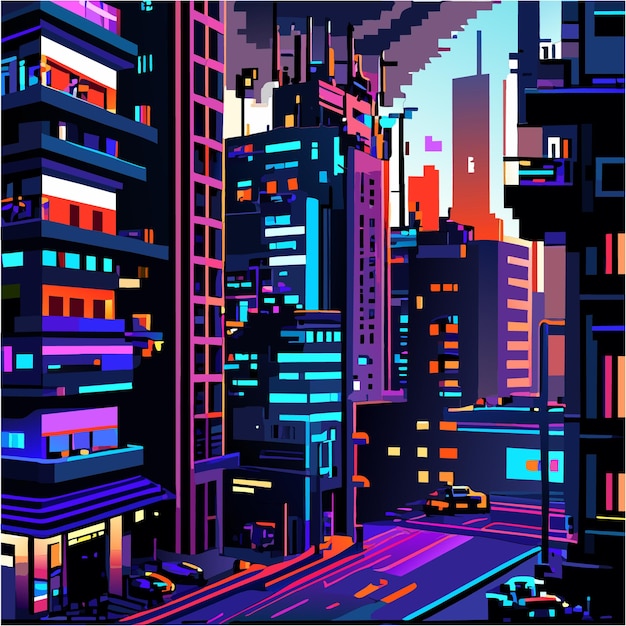The image is a stylized digital graphic depicting a metropolitan area that closely resembles a futuristic New York City. The illustration utilizes boxy, vertical designs to represent high-rises and residential buildings, creating a cartoonish, non-realistic aesthetic. The color palette is predominantly cool, featuring shades of purple, light blue, dark navy blue, pink, and some oranges. The horizon is a tapestry of these colors, with a darker gray area that might suggest clouds. The skyscrapers and buildings have different stories, adorned with windows illuminated by yellow and orange lights, adding depth and vibrancy.

Tall buildings are situated on both the left and right sides, and prominent on the upper portion is a blue sky with a slight gradient and a light pole poking out from one of the buildings. The bottom part of the graphic includes a detailed intersection with purple, pink, and blue roads, populated by a few cars and futuristic-looking motorcycles. There are storefronts on the lower left side, contributing to the bustling cityscape. Overall, the graphic is an artistic, highly stylized rendition of a city infused with a futuristic and almost surreal quality.